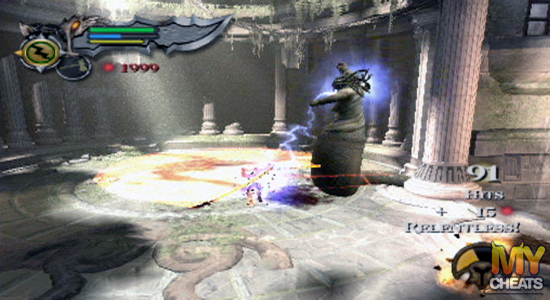The image captures a scene from a video game set within a dilapidated stone castle. The setting's focus is a circular hall adorned with numerous pillars, many of which appear broken or partially crumbled. The structure is ancient, giving off a sense of age and mystery. At the center of the scene stands an enigmatic figure, exuding an aura reminiscent of a Greek goddess, with bolts of blue lightning emanating from her form, adding an ethereal glow to the otherwise somber environment.

The game's interface overlays the scene with various HUD elements. On one side, there is a notification titled "My Cheats," displaying stats which include "91 points plus 15," next to an icon and the word "Reptiles." At the top of the screen, three meters are visible: one green and completely full, one blue and half-full, and one yellow, also completely full.

Ambient lighting indicates that the roof of the castle is either missing or severely damaged, as visible beams of sunlight pierce through the open space, creating a dynamic contrast of light and shadow. The interplay of illumination and darkness intensifies as the image transitions from the bright, sunlit spots to the murkier areas, adding depth and atmosphere to the visual.